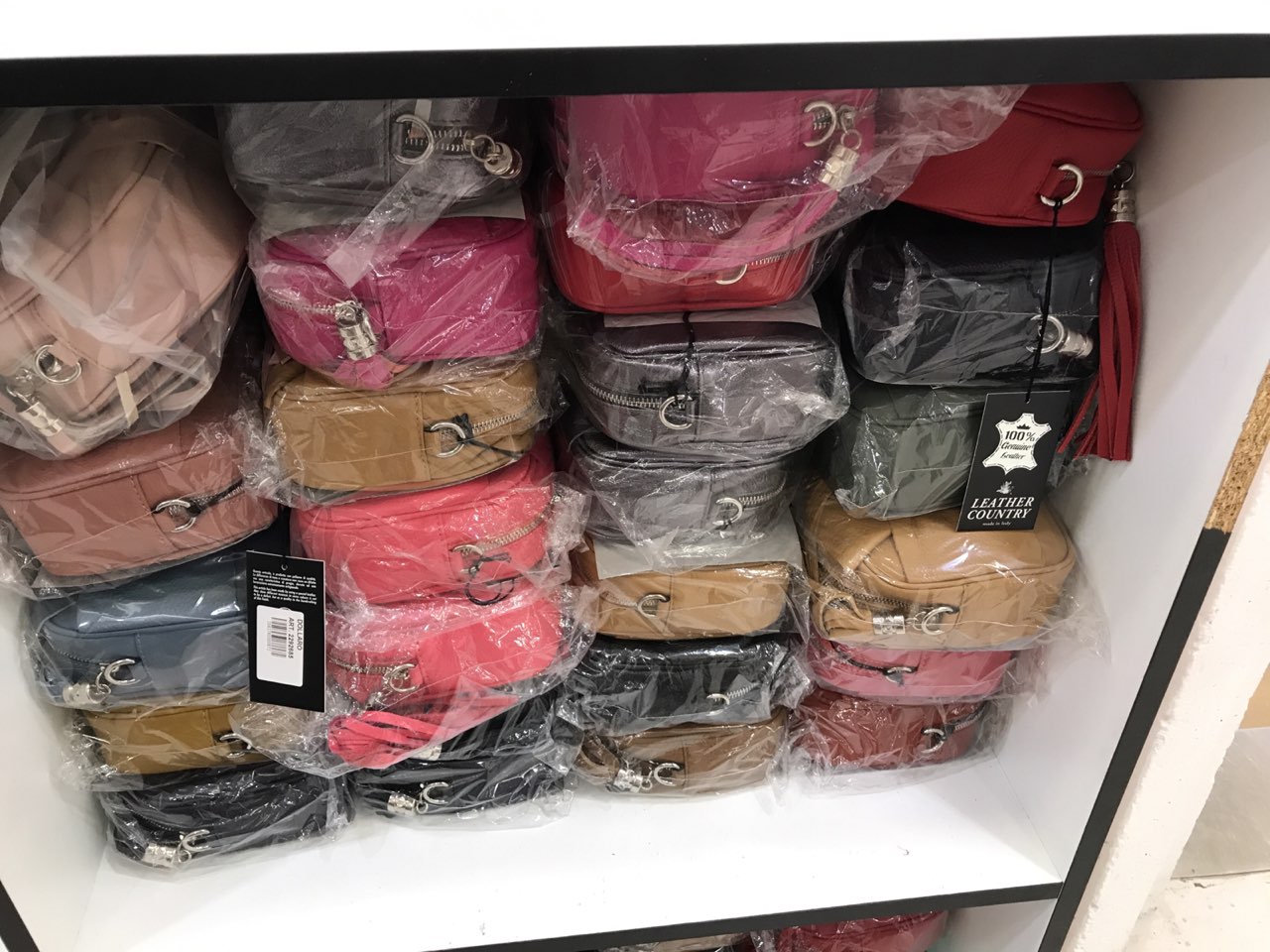This photograph features a white cubby-style shelf taken from a slightly tilted angle. Inside, there are four columns of small leather makeup bags or purses, each column containing a different number of bags: five in the first column, six in the second, seven in the third, and six in the fourth. Nearly all the bags are wrapped in see-through plastic, except for one unwrapped bag in the top right corner. The bags are stacked vertically and display a variety of vibrant colors, including various shades of pink (from light pink to hot pink), coral, salmon, gray, beige, mustard yellow, bright red, black, blue, copper gold, khaki, and a deeper gold. Each bag features a black rectangular tag and some labels indicating their composition as "100% genuine leather." The setup suggests these items are on display in a retail store, neatly arranged and ready for purchase.